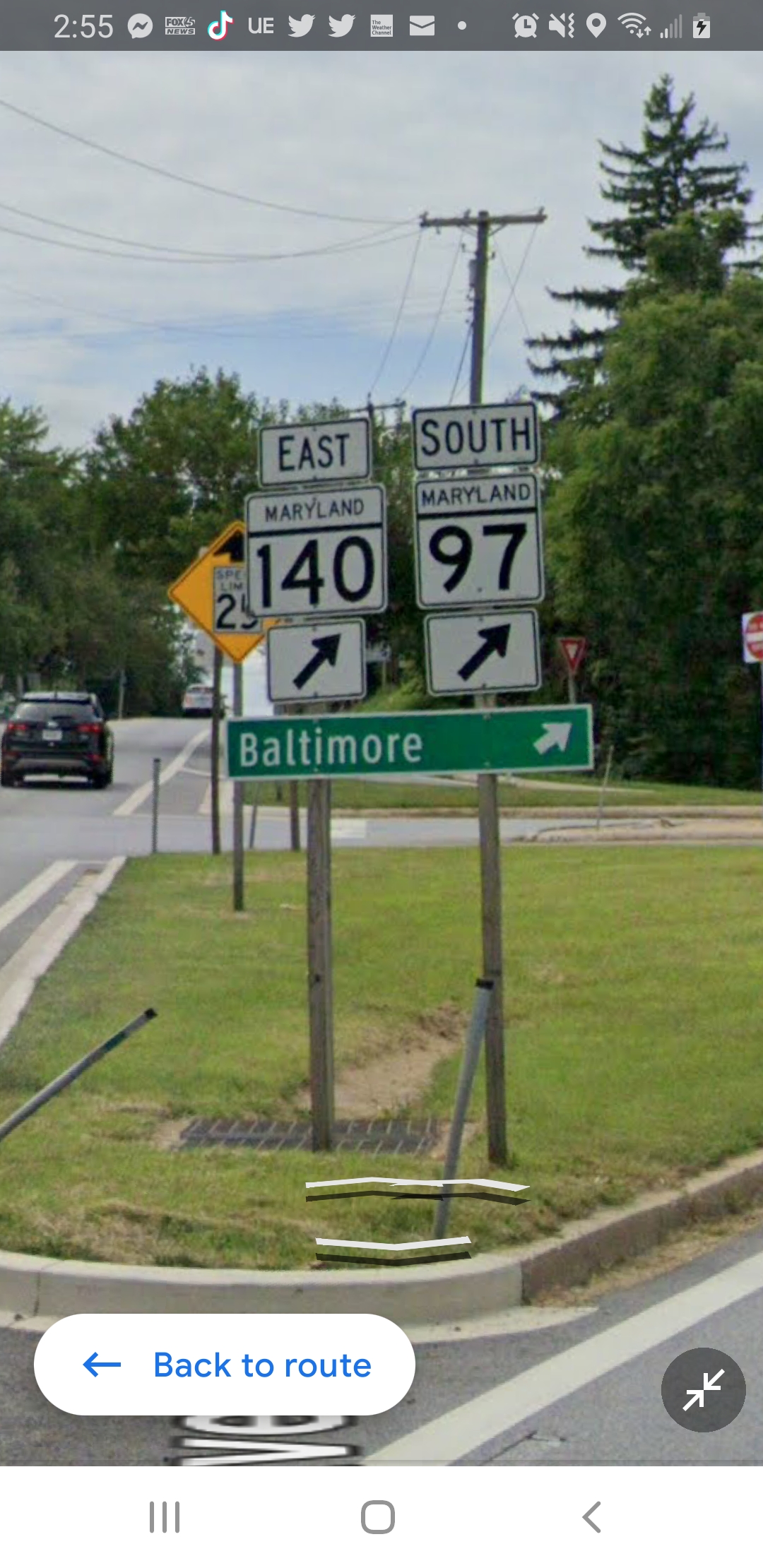The image, likely taken on a smartphone in Maryland, depicts a roadway split by a triangular grassy island. The road diverges, offering options to go straight or curve slightly to the right. Prominent in the scene are multiple traffic signs, inherently instructional, detailing directions and routes. A green sign with white lettering directs traffic towards Baltimore with a right turn, aligned with additional black and white signs indicating East Maryland 140 and South Maryland 97, both with right arrows. Supporting these signs are two wooden poles, possibly replacements for the original metal ones, suggesting prior damage. Overhead cables stretch across the background, amidst tall trees. Two cars are visible on the left road veering leftward, and a distant yellow sign indicates a speed limit of 25 mph. The smartphone interface shows various notification icons at the top, including battery life and signal status, adding to the context of the captured moment.